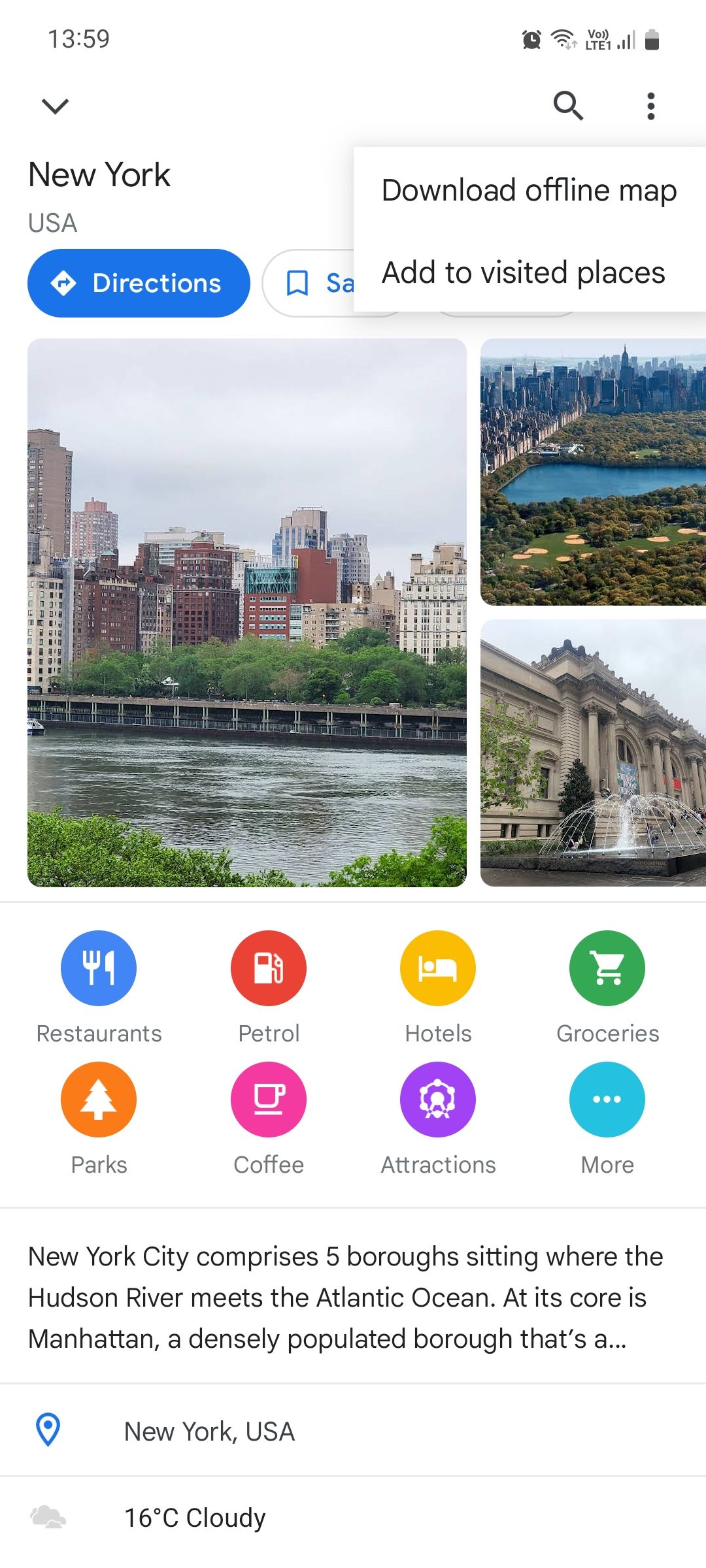The image depicts the screen of a mobile device displaying detailed information about New York, USA. The layout includes several visual elements and icons. At the top of the screen, the time is displayed as 13:59. The central part of the display features a series of images showcasing New York's iconic cityscape, featuring a mix of red buildings, green spaces with trees and grass, and reflective water surfaces. 

Prominent buttons and options can be seen, such as a blue "Directions" button, a "Bookmark" labeled as SA, an option to "Download Offline Maps," and a button to "Add to Visited Places." The upper right corner displays options for exploring various categories like Restaurants, Petrol, Hotels, Groceries, Parks, Coffee, and Attractions, with an additional option labeled "More."

Towards the bottom, textual information summarizes New York's geographical and cultural essence, stating it comprises five boroughs where the Hudson River meets the Atlantic Ocean. The current conditions are also provided, showing a temperature of 16°C and cloudy weather.